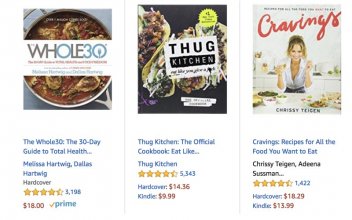Certainly! Here’s a more detailed and cleaned-up caption for the described image:

---

This image showcases three book covers listed for sale on Amazon, each falling within the cooking genre. 

1. **The Whole 30** (Top Left): The book's cover prominently features a crockpot filled with a vibrant red sauce and various ingredients, which immediately convey its culinary focus. The title "The Whole 30: The 30-Day Guide to Total Health," written in blue text, is authored by Melissa Hartwig and Dallas Hartwig. This guide boasts a 4.5 out of 5-star rating from reviewers and is priced at $18. It also features the Amazon Prime logo, indicating fast shipping availability.

2. **Thug Kitchen** (Top Right): Displayed on a stark white square background, bold black text reads "Thug Kitchen." The cover includes enticing images of street tacos set against a contrasting black background. The full title, "Thug Kitchen: The Official Cookbook: Eat Like You Give A F***," suggests an edgy, no-nonsense approach to cooking. This popular cookbook, which also enjoys a 4.5 out of 5-star rating, is available in hardcover for $14.36 and in Kindle format for $9.99, with the price for the Kindle edition highlighted in dark red.

3. **Cravings** (Bottom Right): The book cover presents an inviting scene of a cook (presumably Chrissy Teigen) standing behind a table laden with various dishes, suggesting a rich and diverse selection of recipes inside. The title "Cravings: Recipes for All the Food You Want to Eat" is displayed in blue text, authored by Chrissy Teigen and Adeena Sussman. Garnering a 4.5 out of 5-star rating, this enticing collection is priced at $18.29 for the hardcover and $13.99 for the Kindle edition.

---